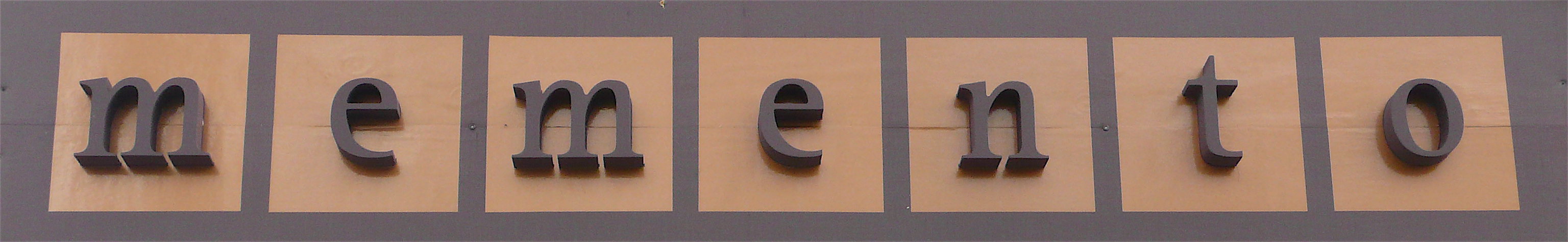The image depicts the name of a store, "Memento," presented in a stylized manner. The store's name is showcased against a dark brown background, adding depth to the overall visual. Each letter, in lowercase, is displayed within its own lighter brown square, reminiscent of Scrabble tiles. The letters are not merely printed on the surface but are raised, giving a three-dimensional effect that adds sophistication to the signage. The arrangement of the tiles, coupled with the choice of warm brown tones, creates a visually appealing and somewhat nostalgic aesthetic. This isolated depiction of the store name against a plain white background emphasizes the unique design and craftsmanship of the store's signage.